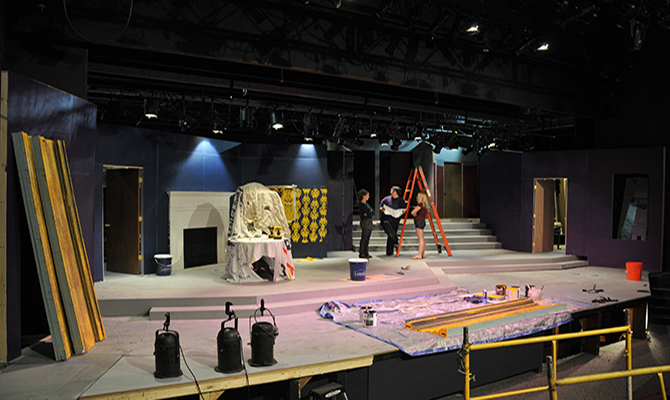The image depicts an unfinished theater stage set in the process of assembly, suggesting ongoing preparations for a stage play. The foreground reveals a clutter of tools and materials: several paint buckets with brushes, wooden boards leaning against the left wall, and a cloth laid out, likely being painted. Three stage lights rest idle on the ground, also to the left. In the center of the stage, a room set takes shape against a dark blue wall adorned with elements like a white fireplace, an ornate orange wallpaper section, and a doorway to the left of the fireplace. A table draped in a white cloth sits in front of the fireplace. In the right section of the stage, near an orange ladder, stand three individuals—one man holding folded papers flanked by two women. This area is characterized by white steps that span from left to right and lead up to a white platform, enhancing the stage’s depth. Above, the rigging for lighting is visible. Overall, the scene is bustling with the activity of preparation, bringing a sense of anticipation for the finalized production.